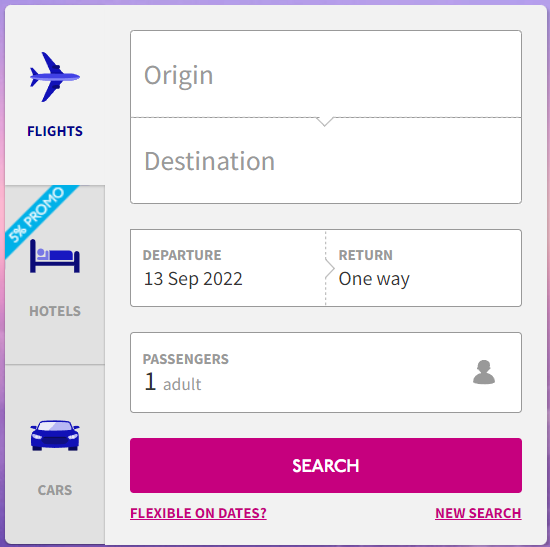Category: Websites

A small interface featuring a light gray background accented with a purple border. In the top-left corner, there's a blue airplane icon labeled "Flights." Directly below it, there is a dark gray square with a teal banner displaying "5% promo," and an icon of a bed representing "Hotels." Further down, the section labeled "Cars" includes a detailed blue car icon, showing the windshield, headlights, side view mirrors, and parts of the tires. On the right side of these icons, the interface consists of a series of white input boxes: at the top is one labeled "Origin," followed by "Destination" underneath it. Below these boxes, another white field is provided for "Departure," set to 13 September 2022, with options for "Return" or "One way," and below that, "Passengers," currently set to one adult.